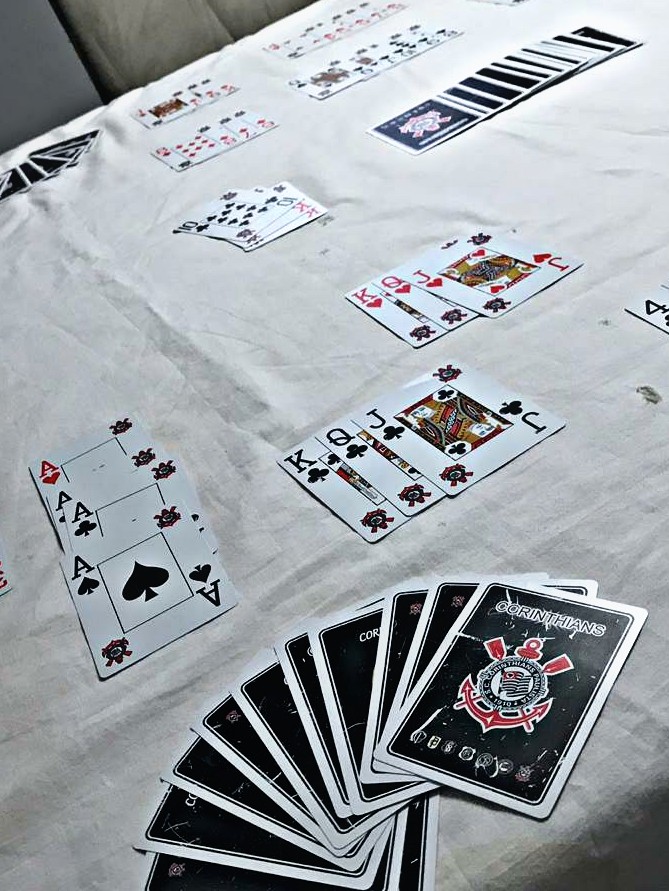On a table covered with a white, slightly wrinkled tablecloth, a diverse array of playing cards is scattered across the surface. In the bottom right corner, a selection of cards is meticulously fanned out in an arch. These cards have a distinctive black background, with the word "Corinthians" emblazoned at the top. Below this title, a black circle frames a red anchor, accompanied by various white icons at the bottom.

To the left side of the table, a neat pile of four cards showcases the different aces. The stack starts at the bottom with the Ace of Spades, followed by the Ace of Clubs, the Ace of Diamonds, and topped with the Ace of Hearts. Intricately arranged just to the right of this pile, three cards are stacked on top of each other, presenting the King of Clubs, Queen of Clubs, and Jack of Clubs in that order. Above this trio, in the center of the table, three additional cards are aligned: the King of Hearts, Queen of Hearts, and Jack of Hearts.

Further up, a collection of cards with the same black label is spread out, adding to the organized chaos. In the upper left section, close to the center, another interesting arrangement of cards features the Ten of Clubs on top, partially obscuring two other Ten cards. Above this setup, more cards are splayed out, completing the intricate display on the table.